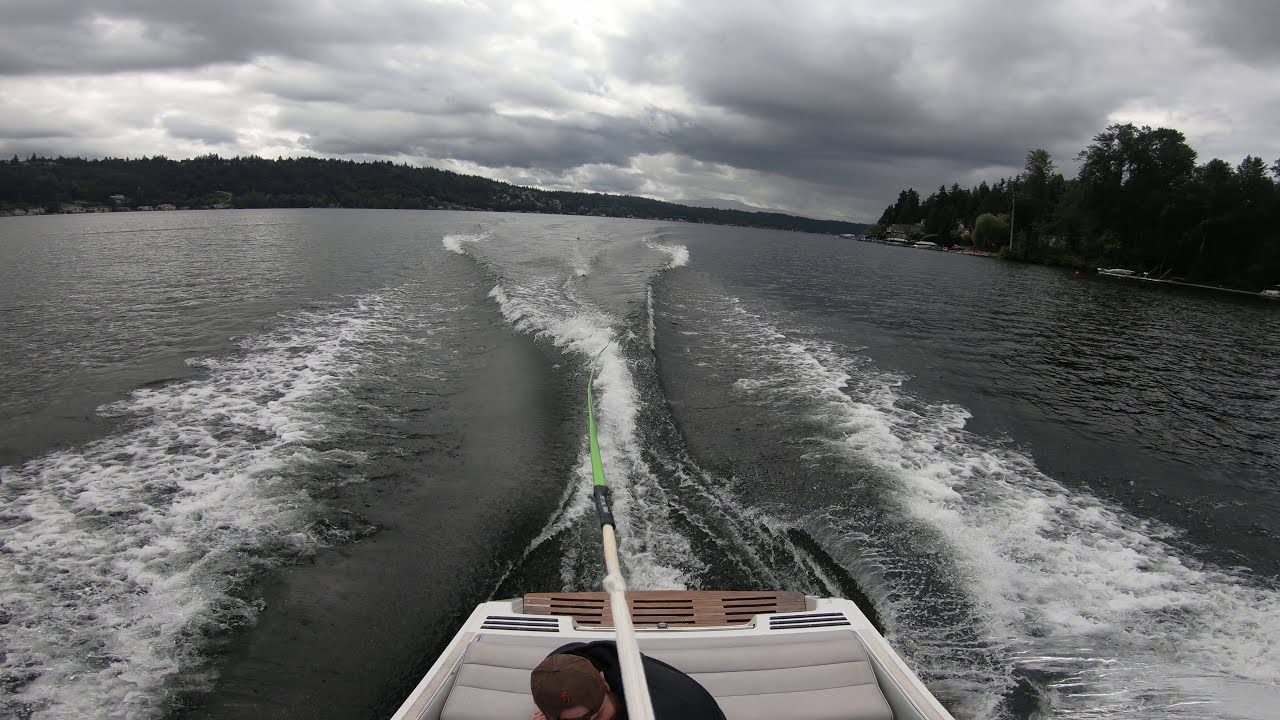The image captures the back of a small, gray and brown motorized boat navigating through a body of dark blue water, creating white-capped waves in its wake. The boat is centrally positioned, filling the bottom third of the image, with a piece of rope colored white, black, and lime green trailing behind it. A man, discernible by his black shirt and brown hat, can be partially seen from the back, primarily showing his head and shoulders. The background features lush green trees sporadically appearing on both the left and right sides, with the right side also showing some rocks and what seems to be a dock with small boats and a shack-like building. The top quarter of the image is dominated by a cloudy gray sky, giving the scene a gloomy, overcast ambiance. The setting suggests a casual boat outing, possibly interrupted by the absence of a wakeboarder implied by the dangling rope.